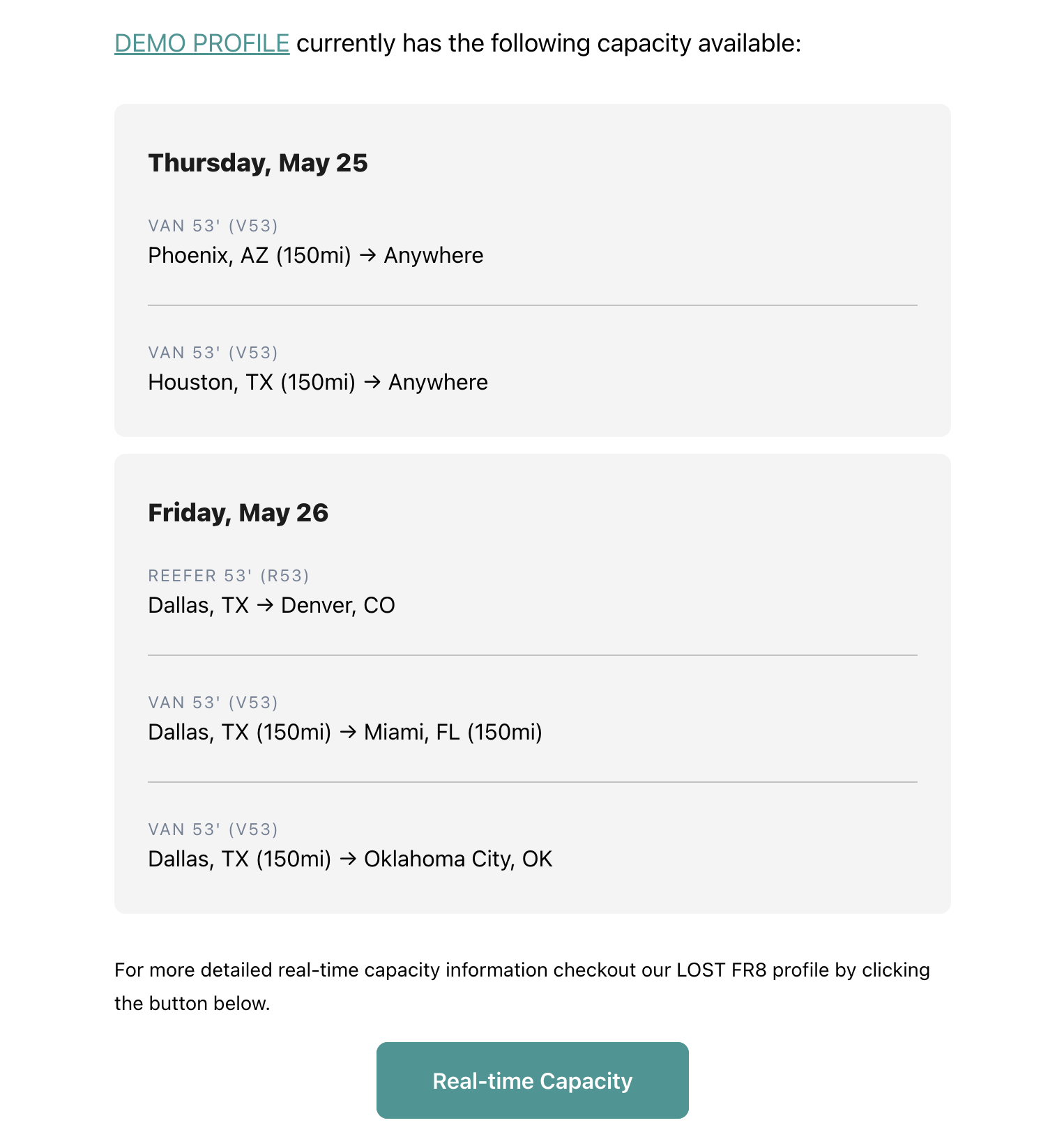The top portion of the image has a white background. Below that, in green, the text "Demo Profile" is underlined. Following this, in black text, it reads, "Currently has the following capacity available:".

The image features two gray rectangles summarizing the available capacities. In the first gray rectangle, Thursday, May 25th is indicated.

- Van 53 (V53)
- Phoenix, AZ (150 miles)

A gray line with an arrow points to:

- Van 53 (V53)
- Houston, TX (153 miles)
  
In the second gray rectangle, Friday, May 26th is detailed:

- REEFER (R53)
- Dallas, TX 

A gray line with an arrow points to:

- Denver, CO 
  
Following that, again for Van 53 (V53):

- Dallas, TX (150 miles)

An arrow points to:

- Miami, FL (150 miles)
  
Lastly, the same Van 53 (V53):

- Dallas, TX (several miles)
   
An arrow points to:

- Oklahoma City, OK